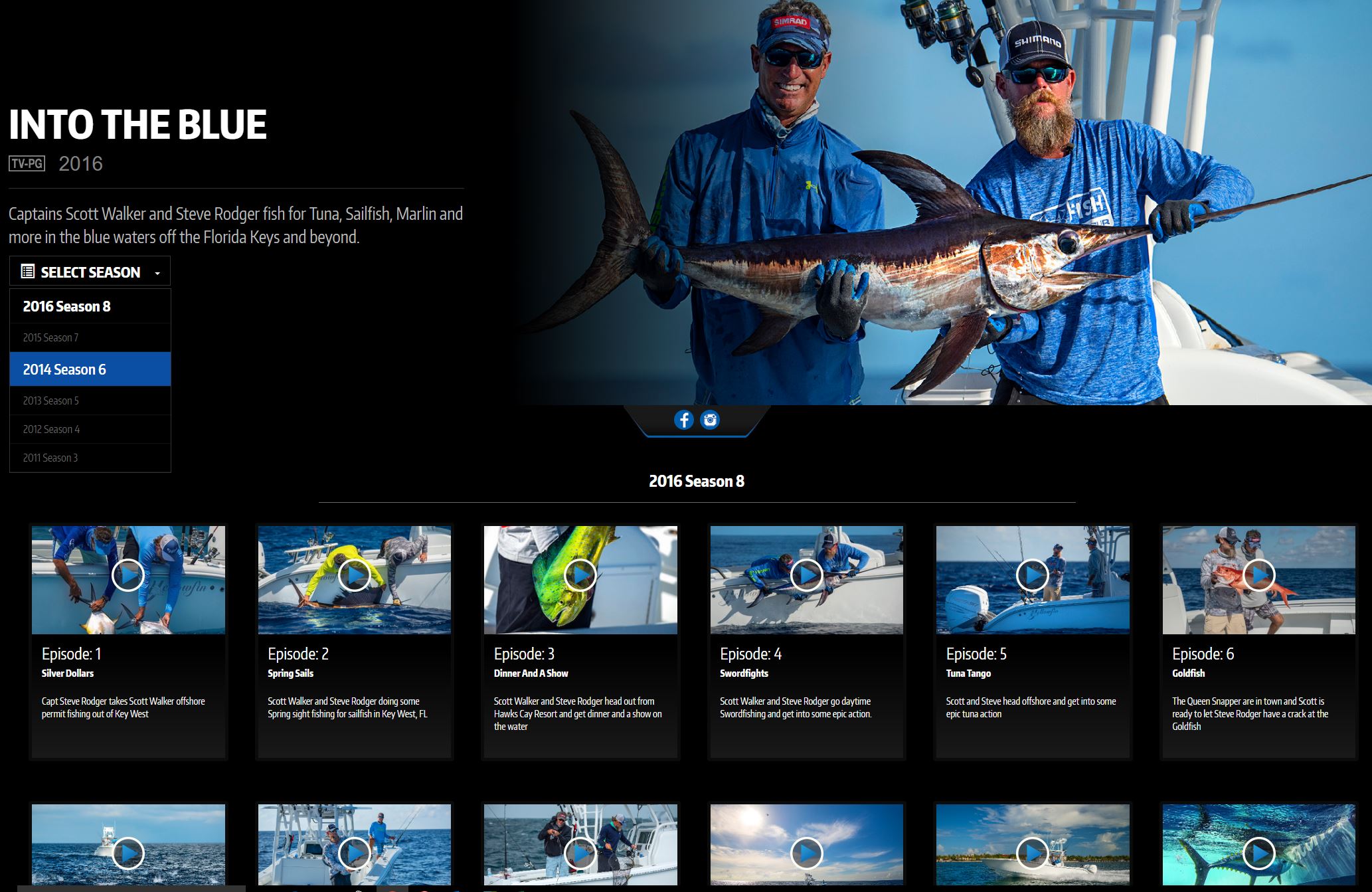This is a detailed caption for an image from a movie streaming website. The layout features a predominantly black background, which occupies the right side of the image and extends halfway down and a bit over halfway across. On the left, there is a clear photo of two men standing outdoors, both dressed in blue, long-sleeve shirts, and wearing black gloves. They are holding a fish horizontally, with its tail oriented to the left and its head to the right. The fish has a long, pointy nose, a black top, black tail, and black fins underneath, while its upper body is white with black eyes.

Both men in the picture are wearing sunglasses and hats. The man on the right sports a beard. The backdrop behind them shows a vibrant blue sky on the right. The background text is in bold, uppercase letters in blue, with the rating TV-PG displayed in gray text below, followed by "2016" also in gray. Underneath this, the caption reads "Captain Scott Walker and Steve Rogers Fish for Tuna, Sailfish, Marlin in the waters off the Florida Keys and beyond."

Below the descriptive text, there's a white rectangle with bold text stating "Select Season." To its left is a smaller white square with black lines and the text "2016 Season 8." Beneath this, black-background options list the previous seasons from 2015 season 7 down to 2011 season 3. Notably, the 2004 season 6 option has a blue background, corresponding to the fish's tail above it. There are also Facebook and camera icons present.

At the very bottom, white text again reads "2016 Season 8," and a row of clickable episode thumbnails is displayed, labeled from episode 1 to episode 6. Each thumbnail includes an image of the men fishing, the episode number, episode name, and a short description. An additional row of six more episode thumbnails is partially visible at the bottom of the image.